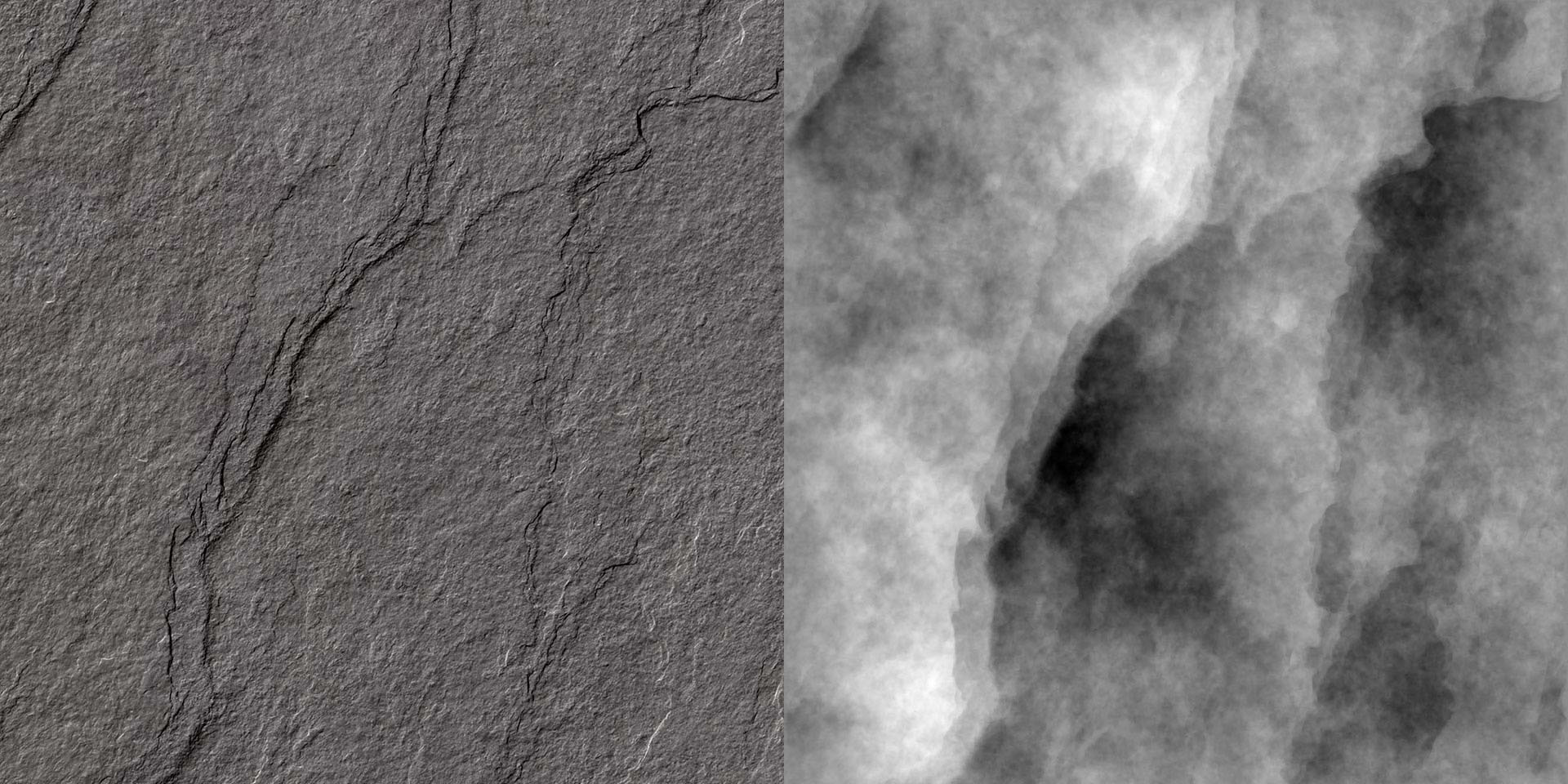This combined image showcases two juxtaposed black-and-white photographs in a square format, positioned side-by-side in a landscape orientation. The image on the left features a close-up view of a rugged gray rock face. It is highly detailed, revealing granular textures, bumps, crevices, and numerous cracks or channels running through the surface. Some darker lines and black cracks also add depth and detail to this striking depiction of natural stone. In contrast, the image on the right presents a more diffuse and ambiguous scene, which could be interpreted as a close-up of clouds, smoke, or a similarly textured surface. This side is characterized by a lighter gray palette punctuated by areas of light and dark, giving it a ghostly, almost ethereal appearance. The soft, puffy textures resemble clouds hovering over hills, adding an abstract and atmospheric quality to the composition. Both images exhibit a harmonious blend of natural elements, unified by their monochromatic color scheme and intricate textural details.